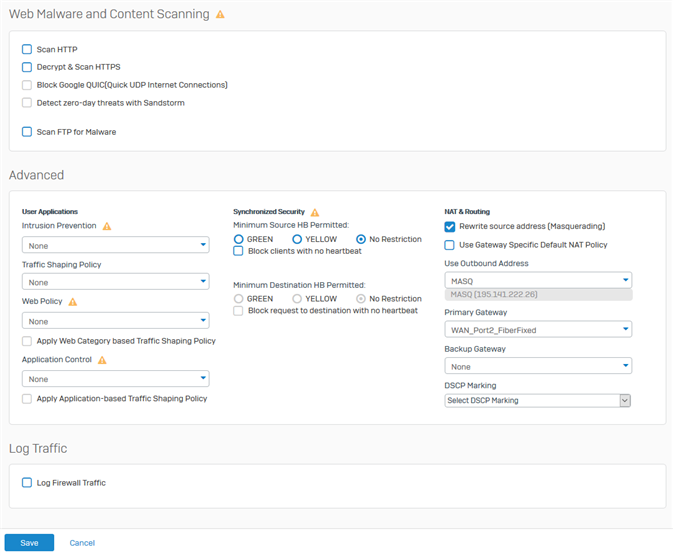This is a detailed and cleaned-up caption for the image described:

"A screenshot of a webpage featuring a predominantly white and gray interface with black text. At the top, it prominently displays the title 'Web Malware and Content Scanning.' Below this heading, there is a yellow triangle icon with an exclamation point inside, denoting a caution or alert. The interface is divided into multiple interactive sections and buttons. 

In the upper-left corner, there’s a smaller rectangle containing clickable boxes, each labeled with different scanning options. The first box is labeled 'Scan HTTP,' and below it, another box reads 'Decrypt and Scan HTTPS.' 

Following this section, there's a larger rectangle labeled 'Advanced' at the top. Within this area, several options are listed, including 'User Applications,' 'Intrusion Prevention,' 'Traffic Shaping Policy,' 'Synchronized Security,' 'NAT and Routing.' 

At the very bottom of the page, a long, thin white box is labeled 'Log Traffic,' with an option below to 'Log Firewall Traffic.' In the bottom-left corner of the screen, there is a small blue rectangle labeled 'Save,' and to its right, another blue text option labeled 'Cancel.'"